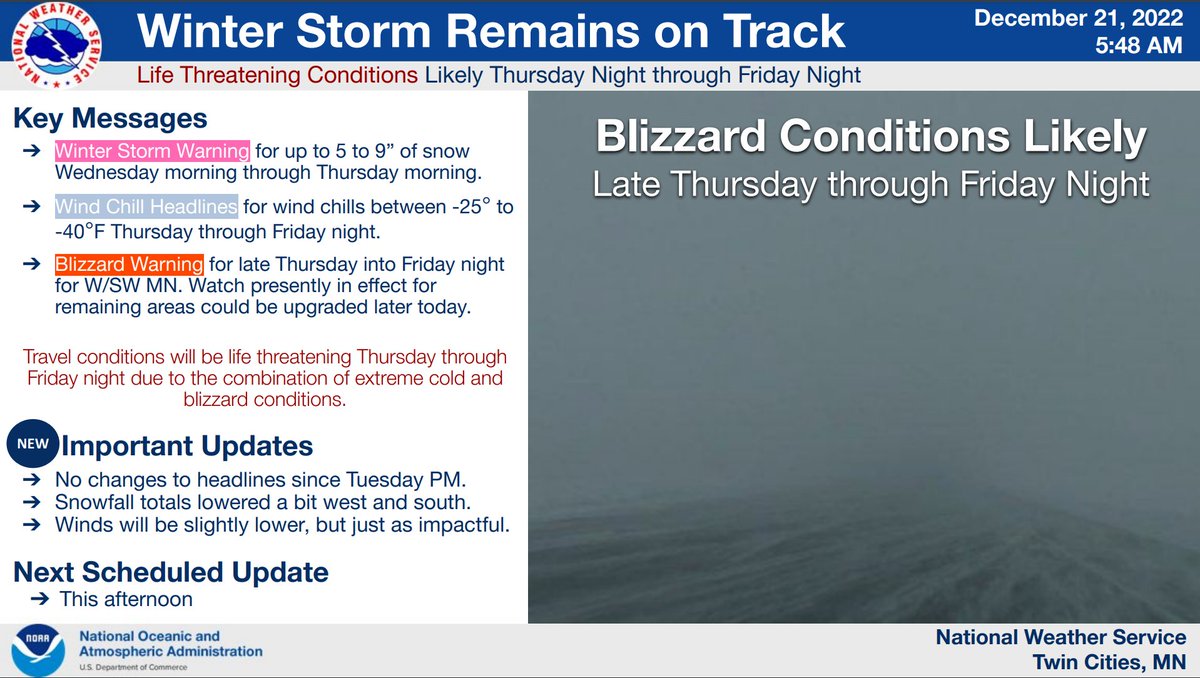**Detailed Caption:**

The image displays a detailed weather advisory for Minnesota, focusing on a winter storm. At the very top, a blue bar with the National Weather Service icon on the left and text reading "Winter Storm Remains on Track" can be seen. To the right, it is dated December 21st, 2022, 5:48 AM.

Central to the image is a photograph resembling a blizzard, with text overlaying it that states: "Blizzard conditions likely late Thursday through Friday night."

On the left side of the image, a "Key Messages" section provides critical information:
1. A winter storm warning is highlighted in pink, forecasting 5 to 9 inches of snow from Wednesday morning through Thursday morning.
2. Wind chill advisory details indicate dangerous temperatures ranging between -25°F to -40°F, expected from Thursday through Friday night.
3. A blizzard warning is noted for late Thursday into Friday night for the west and southwest regions of Minnesota. A watch is currently in effect for other areas, which may be upgraded later today.

An additional note emphasizes that travel conditions will be life-threatening from Thursday through Friday night due to the combination of extreme cold and blizzard conditions. 

Important updates include:
- No changes to the headlines since Tuesday evening.
- Snowfall totals have been slightly reduced for the west and south.
- Wind speeds are expected to be marginally lower but still highly impactful.
- The next scheduled update is slated for the afternoon.

At the bottom left corner, the image indicates the source: National Weather Service Twin Cities/Minneapolis, Minnesota, and the National Oceanic and Atmospheric Administration (NOAA) logo is also visible.

This caption provides crucial information regarding the impending blizzard affecting Minnesota, highlighting predicted conditions, warnings, and updates.